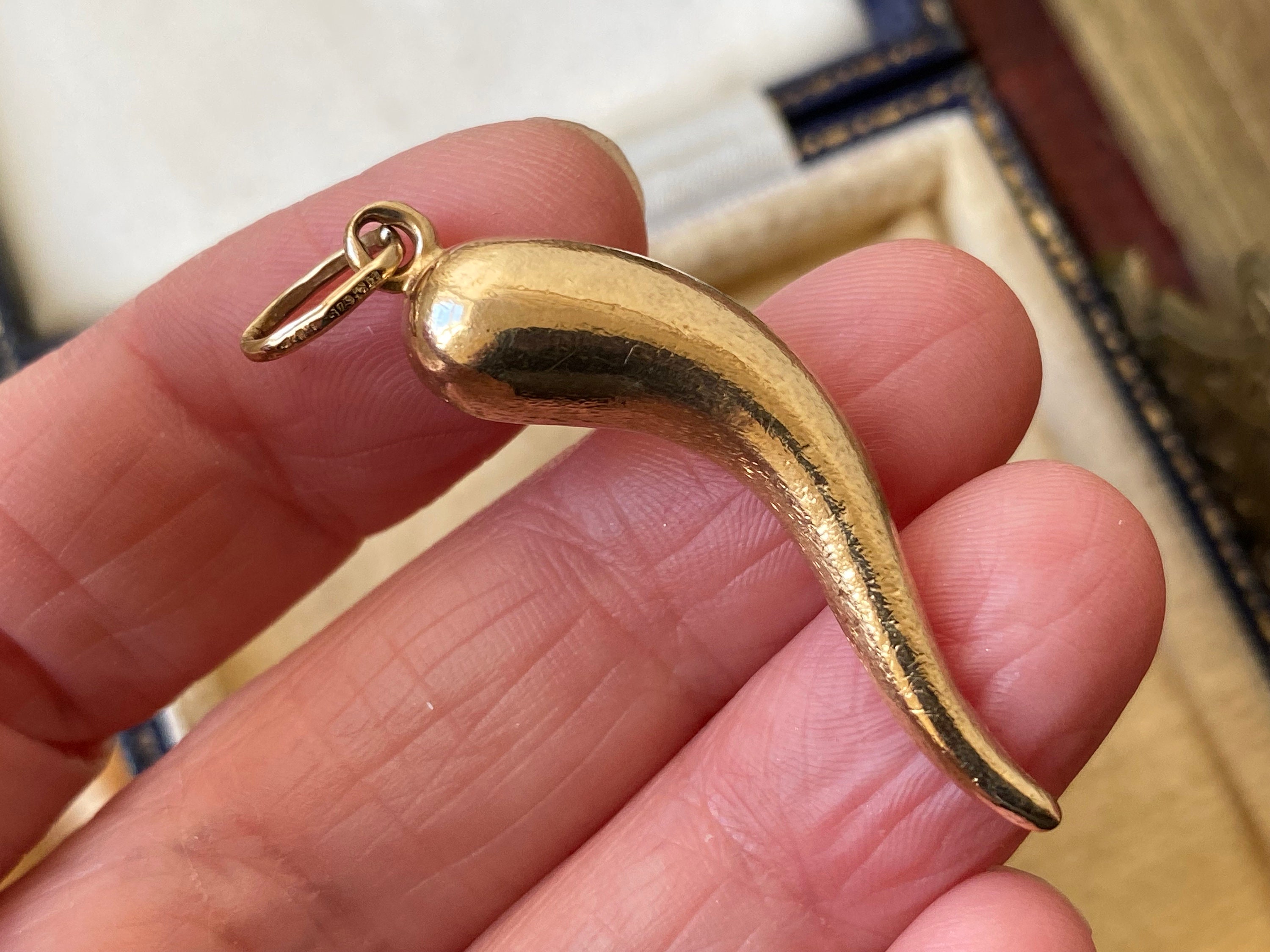The image is a contemporary photograph, slightly wider than it is tall, capturing a close-up of a Caucasian person's hand emerging from the lower left corner. The hand displays the pointer, middle, and ring fingers prominently, with fingers appearing reddish. Held delicately between these fingers is a gold Italian horn charm, reminiscent of the 1980s. The charm, possibly a keychain or necklace pendant, features a characteristic curl and a bail at the top for attachment. The charm appears weathered, with subtle black and white streaks suggesting wear or lighting effects. The background is blurred with colors of cream and brown, and a tray can be vaguely identified, but the focus remains sharply on the detailed hand and the gleaming, vintage charm.